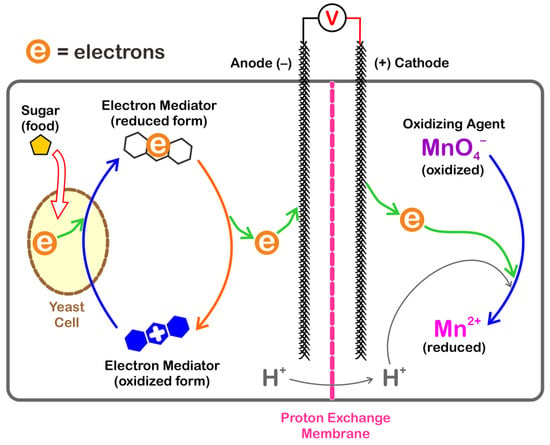The image is an intricate diagram enclosed within a black horizontal rectangle and features a legend at the top left. The legend consists of an orange symbol with the letter "E," representing electrons, and an equal sign. Below the legend is a detailed flowchart visually describing a biochemical process.

The flowchart begins with sugar in food, which enters an oval labeled as a yeast cell, indicating that the process occurs within this cell. From the yeast cell, electrons are transferred to an electron mediator in its reduced form. This mediator then becomes oxidized, with the electrons moving towards the anode – a vertical black and white line on the left side of the diagram, marked with a minus sign.

Next, the electrons proceed to the cathode, which is labeled on the right side of the diagram with a plus sign. The cathode features an associated purple line and an oxidizing agent annotated as "MnO4" in purple letters. Further down, a blue arrow points from "MnO4 oxidized" to "Mn2 reduced," indicating the reduction process.

A key component at the bottom of the diagram is the proton exchange membrane, marked by a dashed pink line, which facilitates the completion of the electron flow. Also noted is an orange "V" symbol near the top, often associated with a voltmeter.

In summary, the diagram depicts the journey of electrons starting from sugar in a yeast cell, through various states and mediators, towards an anode and a cathode, interacting with an oxidizing agent, and concluding with a reduction process facilitated by a proton exchange membrane.